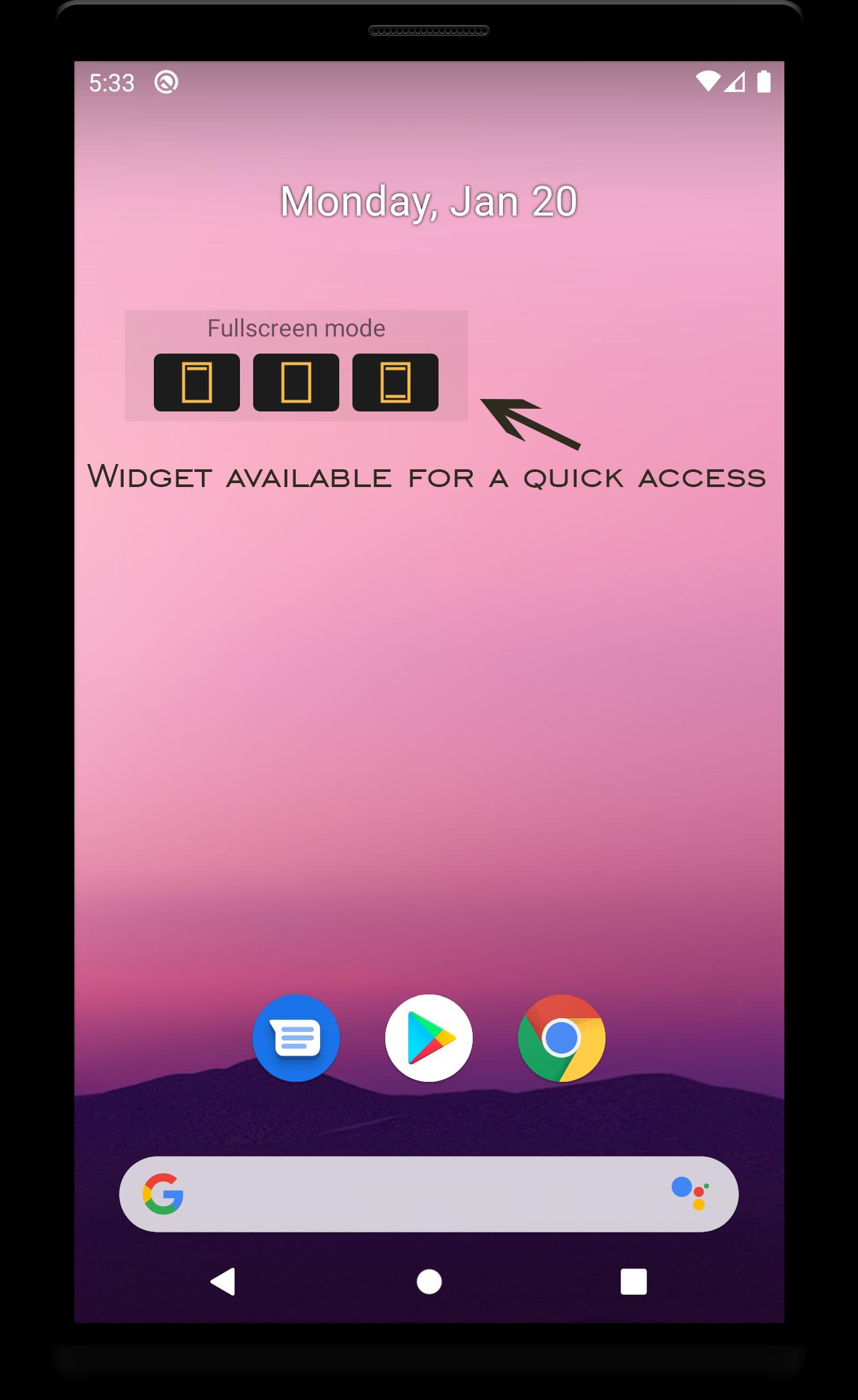The image showcases a smartphone home screen with a primarily light pink background that fades into darker pink and purple hues, mimicking a gentle sunset gradient. At the very top, the date is prominently displayed as "Monday, January 20th", accompanied by the current time in white, and indicators for Wi-Fi signal and battery status. Just beneath the date, a text reads "Widget available for quick access" alongside a black arrow pointing towards a full-screen mode option. This mode features three black icons that likely represent different display options.

The home screen also includes three distinct app logos: 
1. A messaging app icon depicted as a blue circle with white lines through it.
2. A colorful, triangle-shaped logo within a white circle, possibly representing an app store.
3. The recognizable Google Chrome logo, indicative of an internet browser.

At the bottom of the screen, there is a search bar where users can type in their queries. The detailed layout and color scheme of the screen offer an aesthetically pleasing and functional interface.